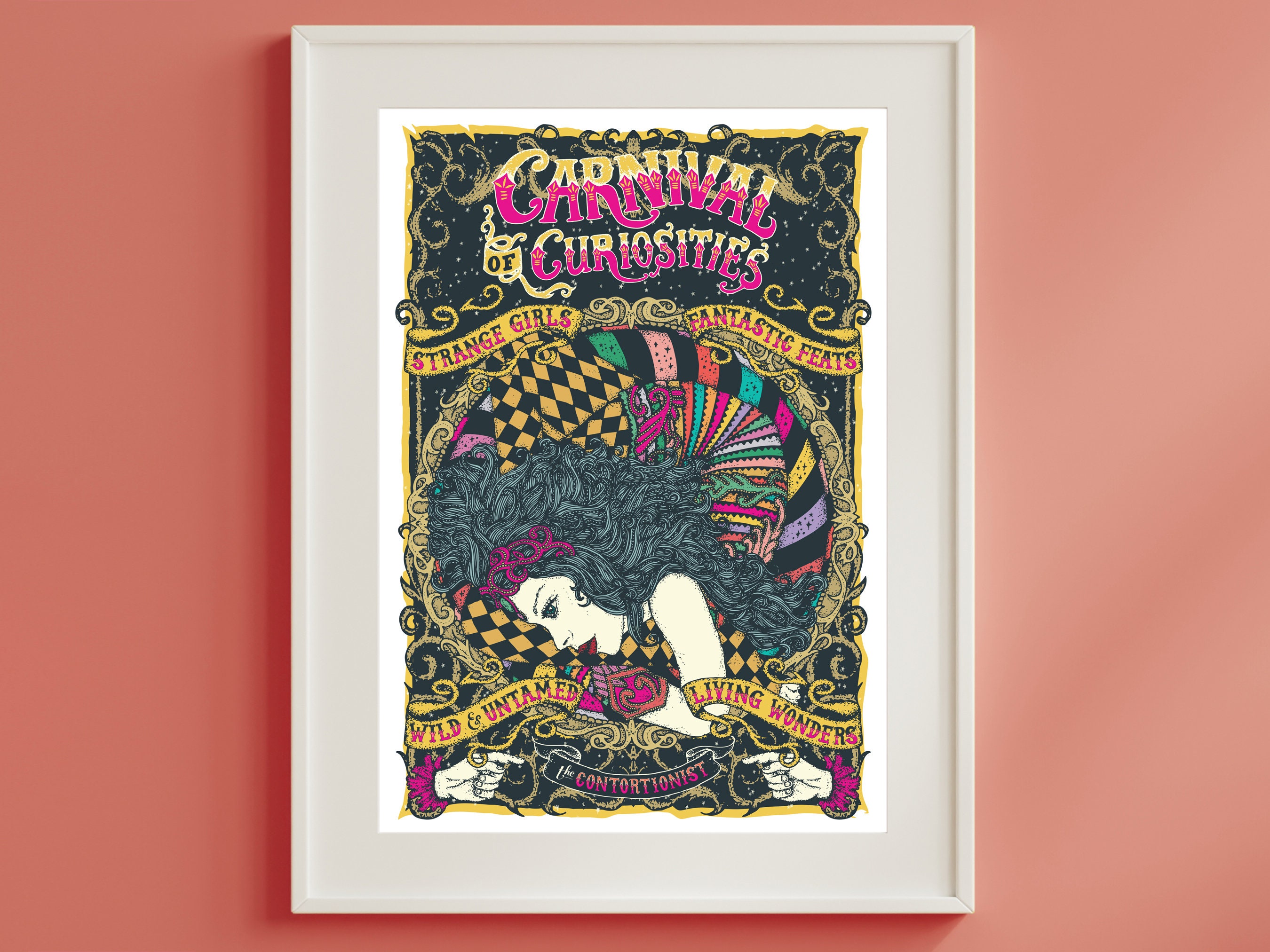This is a detailed photograph of a framed poster, which hangs on a peach-colored wall. The frame of the poster is white, accompanied by a gray mat and a white border around the image itself. The central theme of the poster is "Carnival of Curiosities," depicted in vibrant yellow and pink letters. Within the design, there is a prominent circle adorned with banners that read "Strange Girls," "Fantastic Feats," and "Wild and Untamed Living Wonders."

At the heart of this circle is a drawing of a woman with lush, bushy black hair and pale skin, accentuated by red ribbons in her hair. The detailed artwork utilizes a plethora of colors, including rainbow hues that create a lively and eye-catching background. Additionally, the drawing incorporates various motifs such as cards and branches, enhancing its intricate and busy composition. At the bottom of the poster, two hands clad in pink sleeves point towards the label "The Contortionist," emphasizing this particular act within the carnival theme.